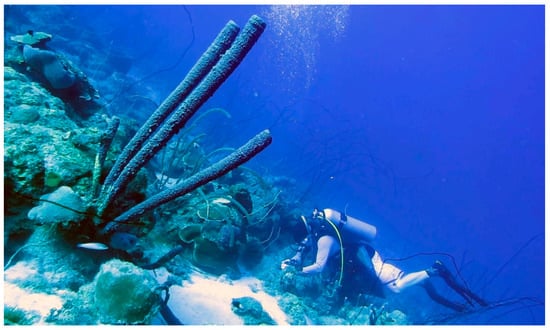This underwater shot captures a mesmerizing scene of an almost unrealistically blue ocean, featuring a solitary scuba diver who appears to be examining or picking something up from the seabed. The diver, positioned centrally at the bottom of the image, is surrounded by vibrant coral and large sea sponges, predominantly shaded in green and blue, set against a white sandy or rocky area. The left side of the image reveals a variety of rocks, coral, and plant life, including reed-like structures. The diver is equipped with black fins, a silver oxygen tank, and a green tube running from the tank to the front. Notably, the diver is not wearing a full-body wetsuit, allowing a clear view of their arms as well as their legs, including defined calf muscles. A field of bubbles extends upwards from the diver, enhancing the realism and dynamic nature of the photograph, which vividly showcases the underwater world in meticulous detail.